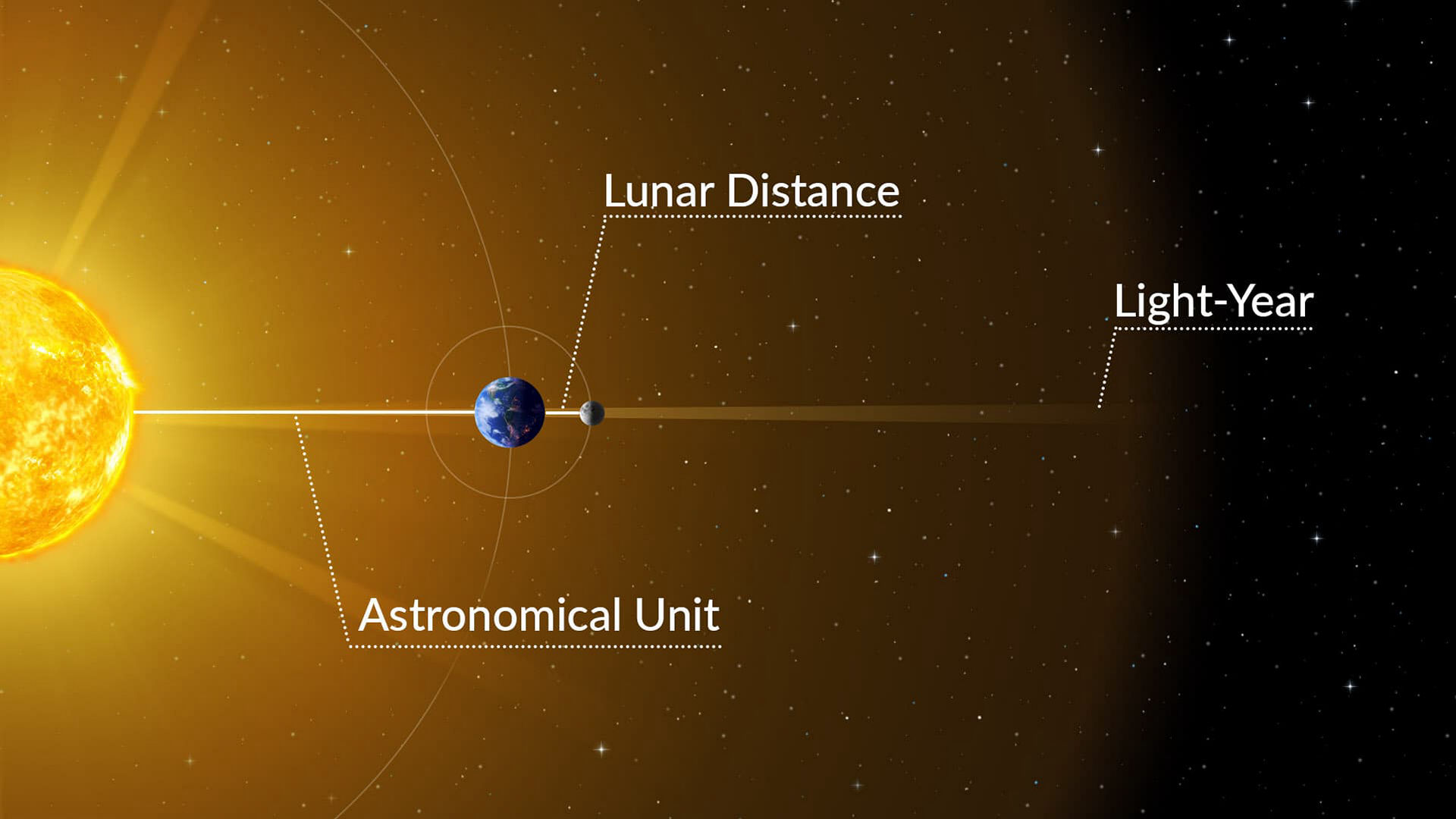The image depicts a detailed view of outer space, primarily showcasing distances within our solar system. On the left, there is a prominent, bright yellow circular celestial body, the Sun, radiating an intense yellow light with darker orange areas on its surface, accentuated by a glowing golden lens flare effect. Surrounding the Sun is a faint circle representing its influence. To the right of the Sun, a line labeled 'Astronomical Unit' extends towards the outer regions of the image; this line is further marked with labels, including 'Lunar Distance' to indicate the distance to the Moon. The sky gradually darkens from left to right, transitioning from the Sun's bright glow to the black expanse of space dotted with white stars.